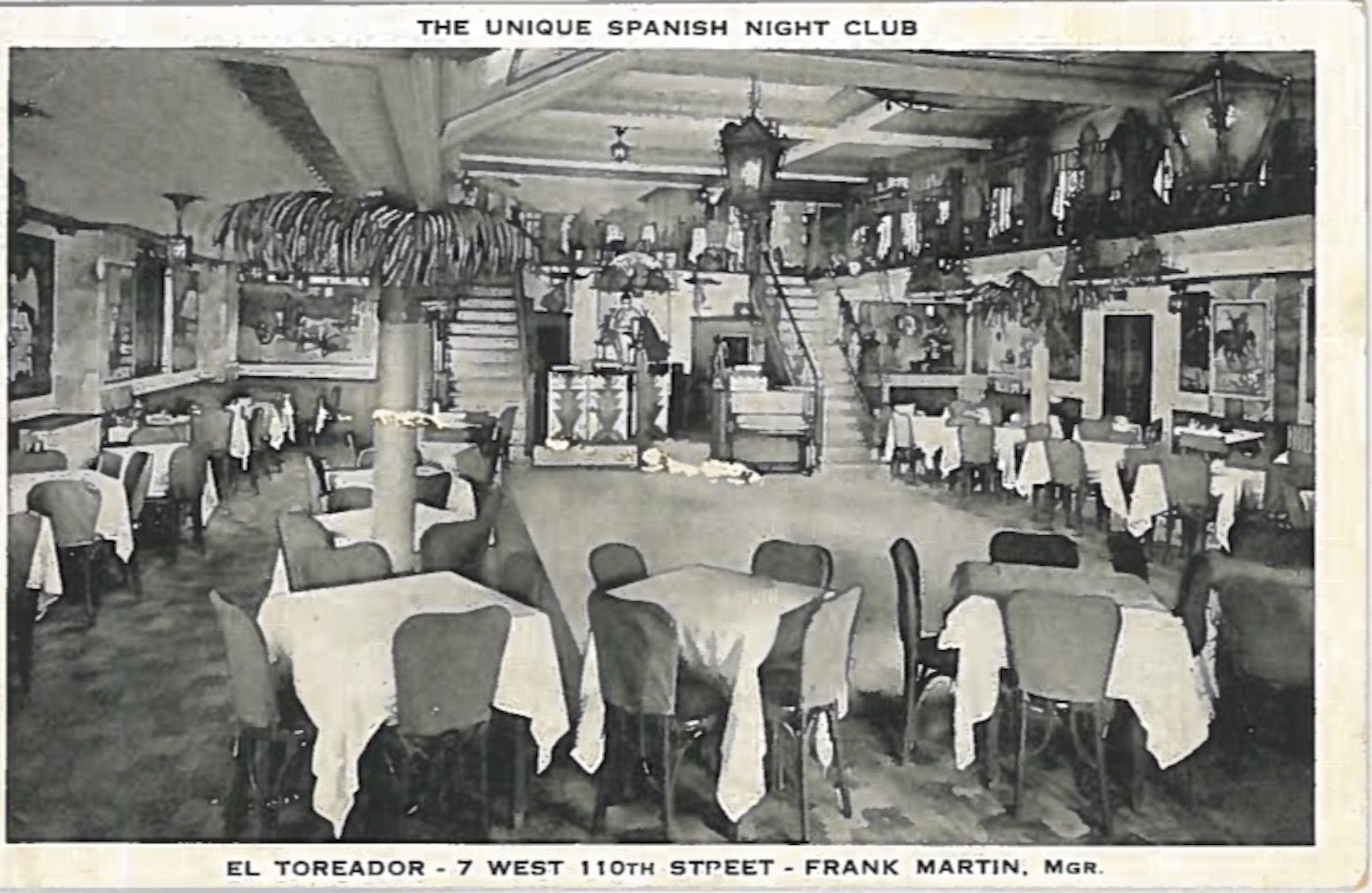This is a vintage black-and-white photograph of the dining room inside a historic restaurant and nightclub, labeled "The Unique Spanish Nightclub." The sign at the top reads "The Unique Spanish Nightclub" and at the bottom, "El Toreador, 7 West 110th Street - Frank Martin, MGR." The room is filled with numerous square tables, each draped in white tablecloths and surrounded by four to five chairs, some with seat coverings. The tables are arranged around a central dance floor. The scene is illuminated by black hanging lanterns and old-style chandeliers. In the background, two staircases ascend to a second floor that hosts more tables. A palm tree decorates the left side of the image, adding to the distinctive ambiance of the space.